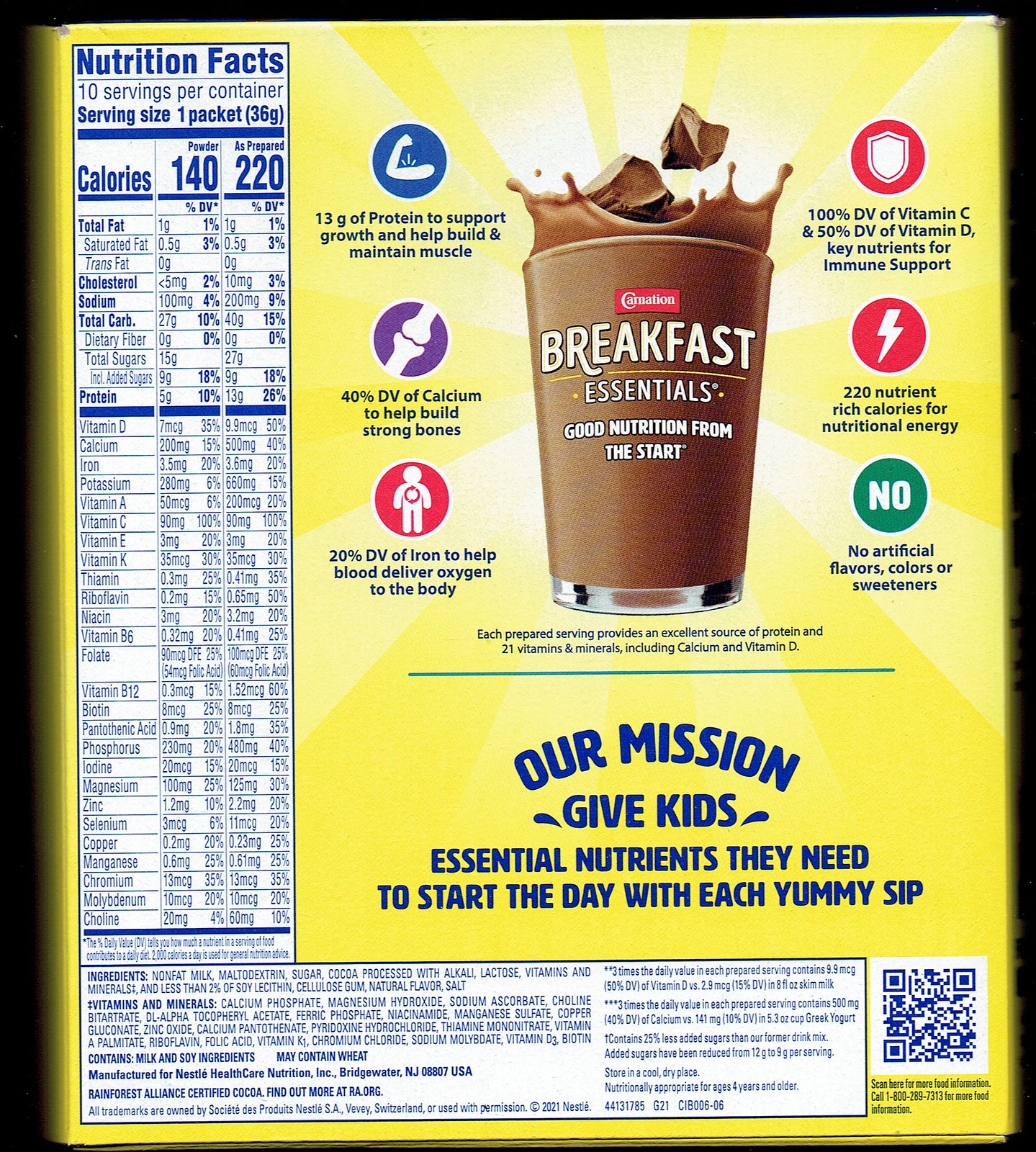The back of the Carnation Breakfast Essentials drink mix box features a detailed Nutrition Facts label on the left, displaying the calories, ingredients, vitamins, and macronutrients. The main section showcases a tempting image of chocolate milk in a see-through glass cup, with chunks of chocolate splashing into the milk. Prominently displayed is the Carnation logo with a red background and white text, accompanied by the tagline "Good Nutrition from the Start." Surrounding the glass of chocolate milk are informative icons detailing the product's benefits: a blue icon boasting 13 grams of protein for muscle support, a purple icon highlighting 40% of the daily value (DV) of calcium for strong bones, a red icon specifying 20% of the DV of iron for oxygen transport, another red icon ensuring 100% DV of Vitamin C and 50% DV of Vitamin D for immune support, an orange icon noting 220 nutrient-rich calories for energy, and a green icon indicating no artificial flavors, colors, or sweeteners. At the bottom right, a QR code is available for additional information. Below the nutrition label, the mission statement reads, "Give kids essential nutrients they need to start their day with each yummy sip." The box contains ten packets of the drink mix, each designed to be mixed into a nutritious chocolate beverage.